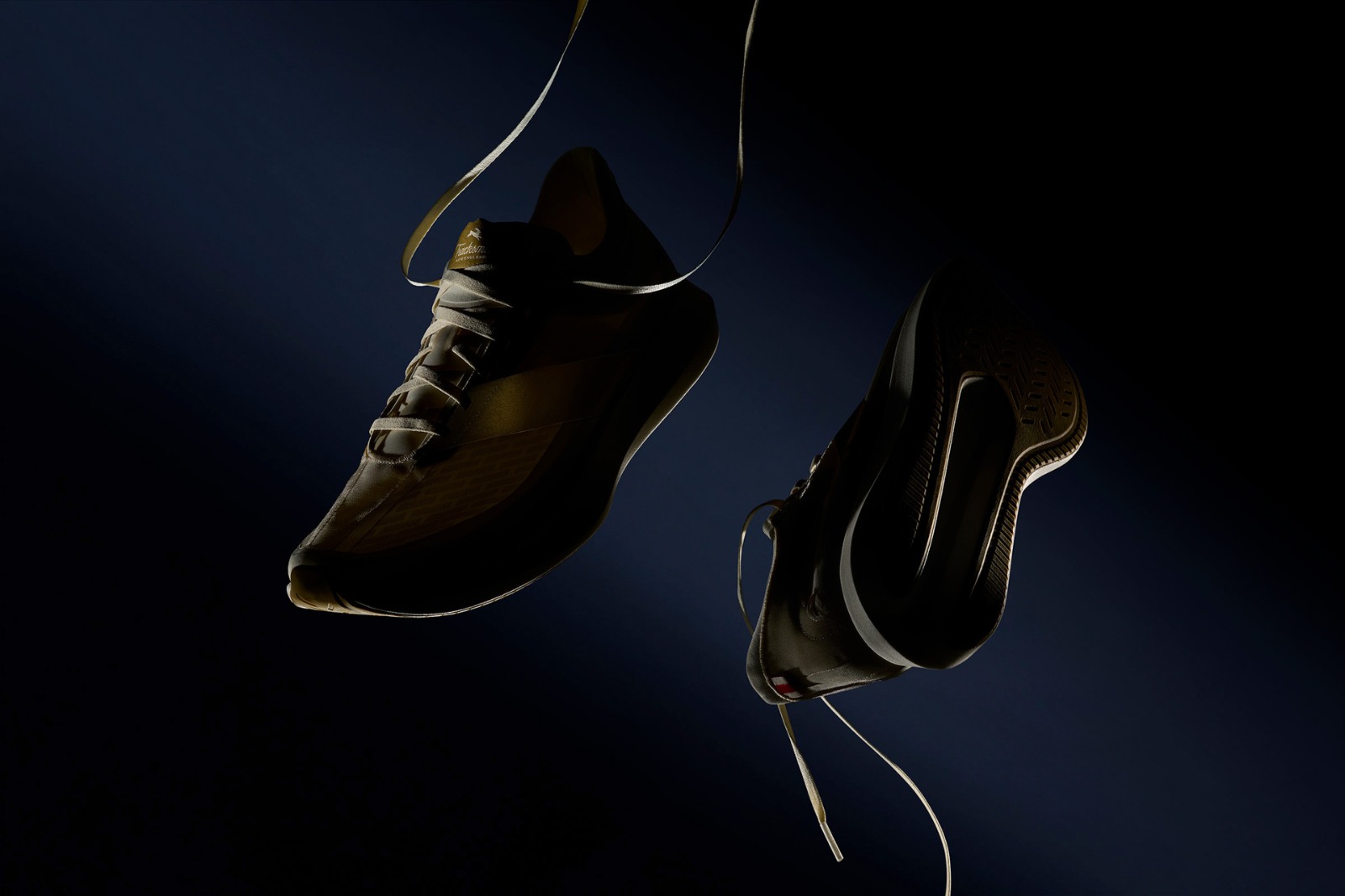The image depicts a pair of floating sneakers set against a predominantly very dark navy blue background. A swath of lighter navy blue runs diagonally from the top left to the bottom right, creating a striking contrast. The left shoe hangs from its white laces at the top of the frame, showcasing its bronzed, black, and shiny leather-like upper. The right shoe, also suspended midair, is turned upside down, revealing its sole and dangling white laces. The sneakers appear almost illuminated, enhancing the metallic sheen on their surfaces. No brand is discernible in the image.